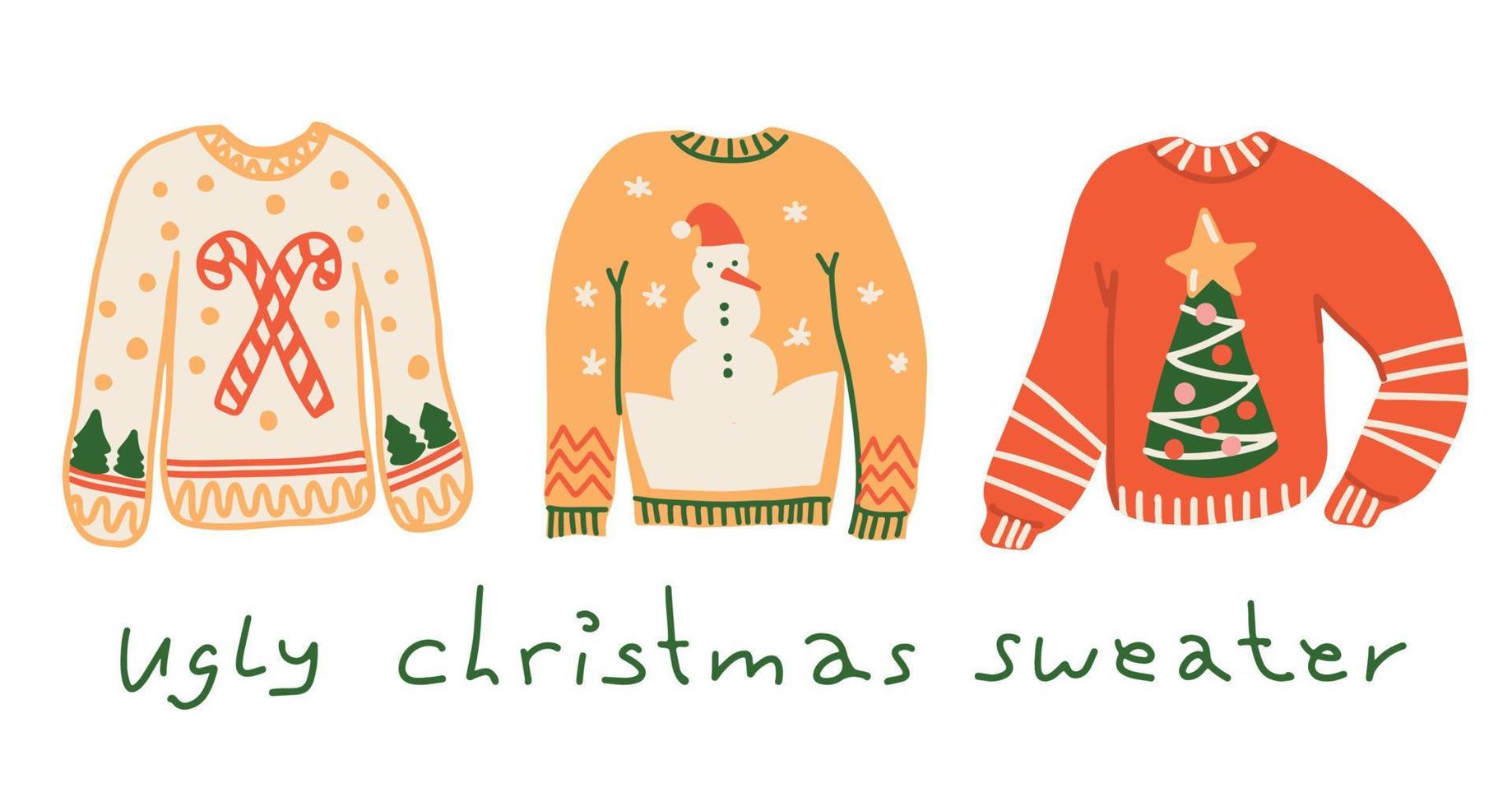The image resembles an advertisement for an Ugly Christmas Sweater party invitation, featuring hand-drawn, cartoonish-style sweaters arranged in a horizontal row. Each sweater is intricately designed and colorfully detailed. 

The first sweater is a light cream color, adorned with crisscrossed candy canes and yellow polka dots. It has yellow zigzag trims around the neck and sleeves, suggesting a mountain-like design. Each sleeve also features two small green fir trees.

The second sweater is a warm, mustard yellow or clementine orange color with a central snowman motif. The snowman, complete with black buttons, a carrot nose, two eyes, and a Santa hat, sits amidst snowflakes. This sweater is trimmed in green at the neck, cuffs, and hem, with red zigzag patterns on the sleeves.

The final sweater is a vibrant orange with a Christmas tree decorated with multi-colored balls in its center and a yellow star at the top. It features white stripes on the sleeves, collar, and hem for added contrast and design. 

Below the trio of sweaters, the phrase "Ugly Christmas Sweater" is printed in green, child-like font, enhancing the playful and festive theme of the image.